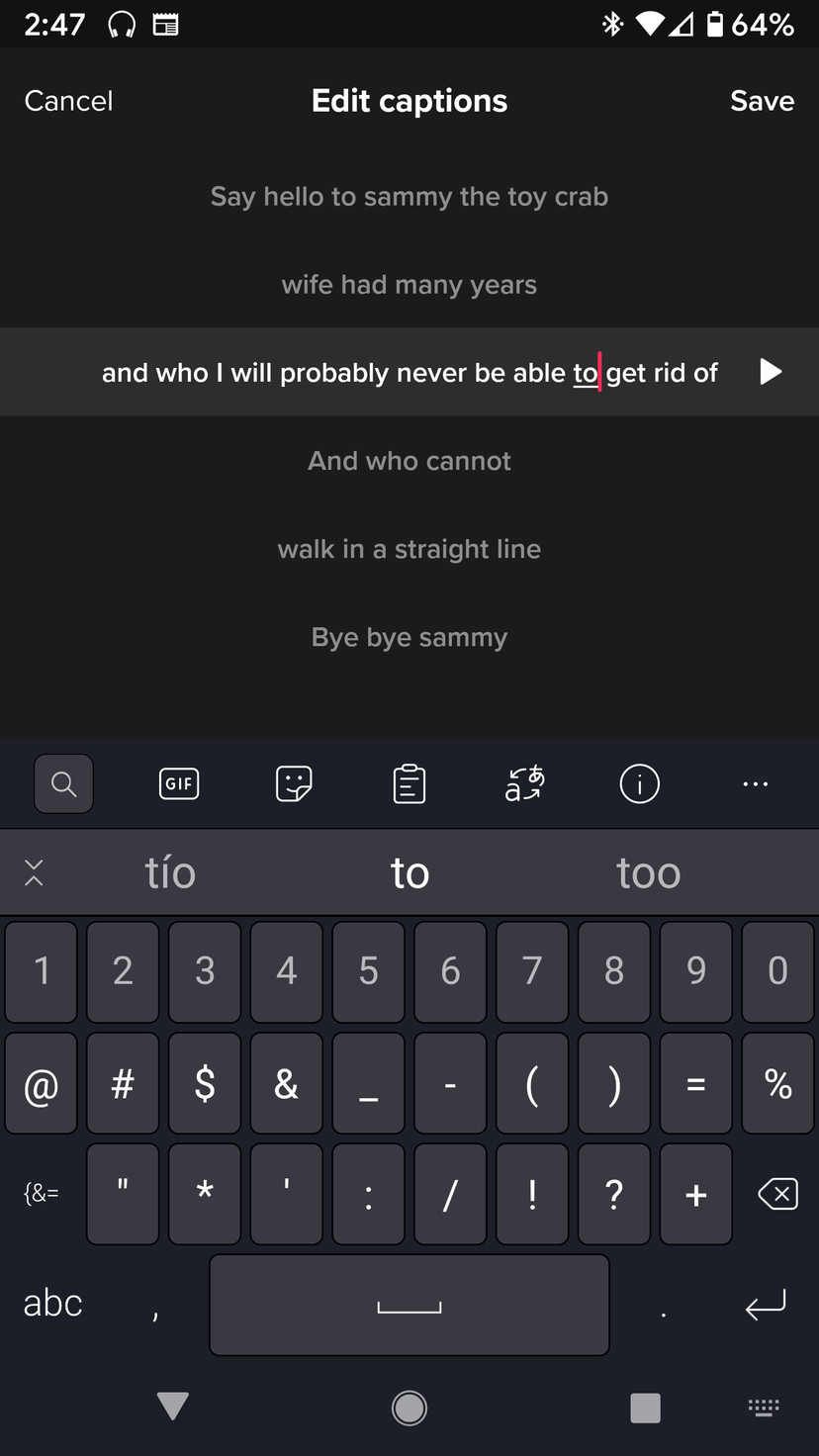Here we have a detailed screenshot from a smartphone interface. At the top of the screen, the status bar displays the time, 2:47, accompanied by a headphone icon, a Bluetooth icon, a Wi-Fi signal icon, and a battery icon indicating a 64% charge. 

Just below the status bar, there is a navigation bar featuring three options: "Cancel" on the left, "Edit Captions" in the center, and "Save" on the right. Under these options, a list of suggested captions is displayed. The list begins with "Say Hello to Sammy the Toy Crab." The next item reads "Wife had many years." The third item, which is highlighted, states "Anne who I will probably never be able to get rid of," with a red line right after the word "to" followed by additional text with arrows and phrases: "who cannot," "walk in a straight line," and "by by Sammy."

Beneath the list, there is another functional row containing icons for search, gift, note, information, and a three-dot menu representing more options. Below this row, a gray text box displays the text "TO2" (T-O, 2 as in T-O-O).

At the bottom of the screen, a virtual keyboard is visible, displaying numbers 1 through 9, 0, and various commonly used symbols like @, &, and $. The keyboard also includes a space bar, an "ABC" option for switching to alphabetical input, a button for correcting mistakes, and a backspace key. Finally, the bottom-most part of the screen features the Android navigation buttons: a triangle (Back), a circle (Home), and a square (Overview).